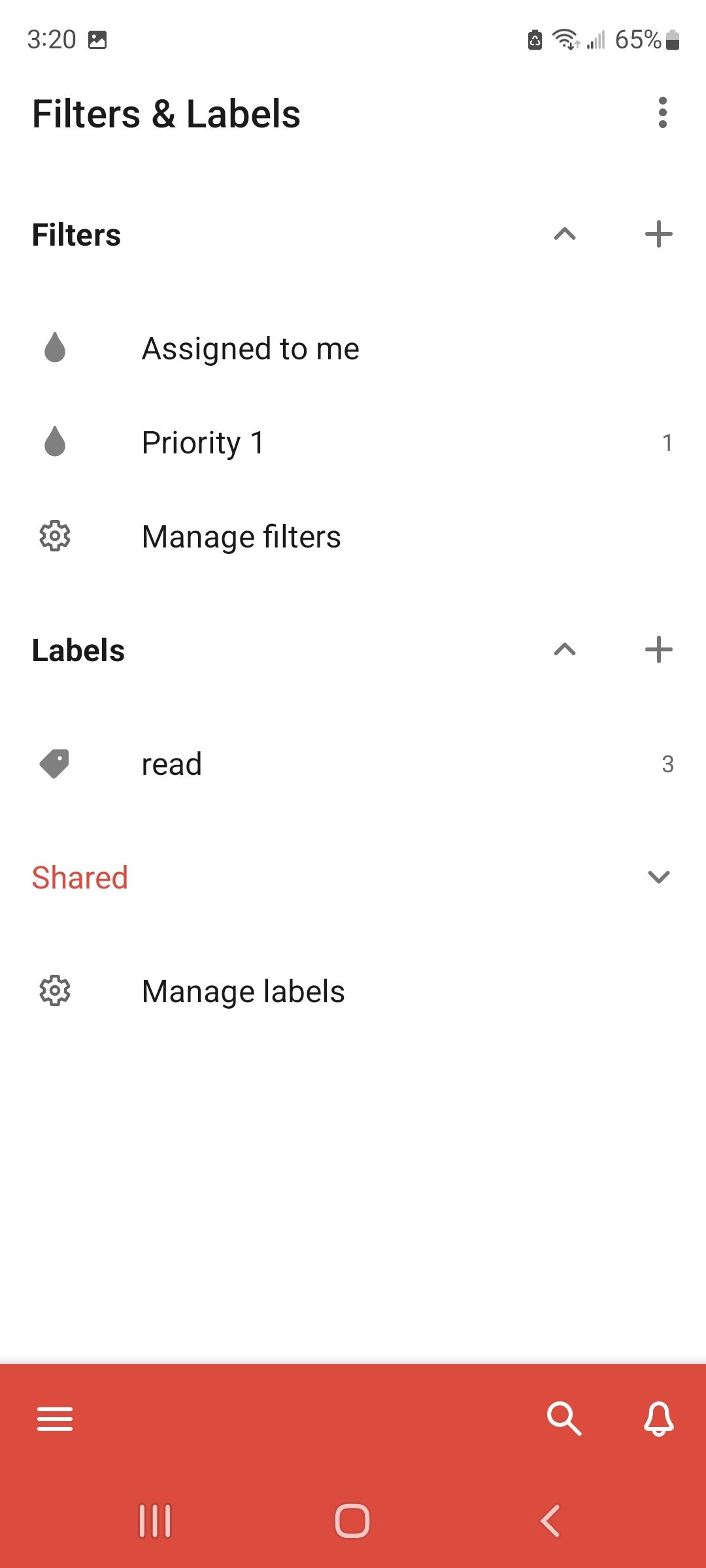This image is a screenshot from a mobile phone. In the upper left corner, the time reads 3:20, and to the right of it is a battery icon indicating 65% charge. On the left side of the screen, there's a section labeled "Filters and Labels" in black text.

Under "Filters," there are three subsections:
1. "Assigned to Me" with a black drop icon beside it.
2. "Priority 1," also accompanied by a black drop icon.
3. "Manage Filters" which features a gear icon.

Next, under the "Labels" section, the following options are visible:
1. A tag icon labeled "Read."
2. A red label titled "Shared."
3. "Manage Labels," which includes a gear icon to its left.

At the very bottom, there is a red rectangle that contains a set of icons. On the upper left corner of this rectangle, there are three horizontal white lines. To the right, there is a magnifying glass icon next to a white bell. At the very bottom of the rectangle, three vertical lines appear in a row beside a white square, followed by a left-pointing arrow.

The interface appears to be user-friendly, providing organized options for managing and filtering various tasks or messages on the device.